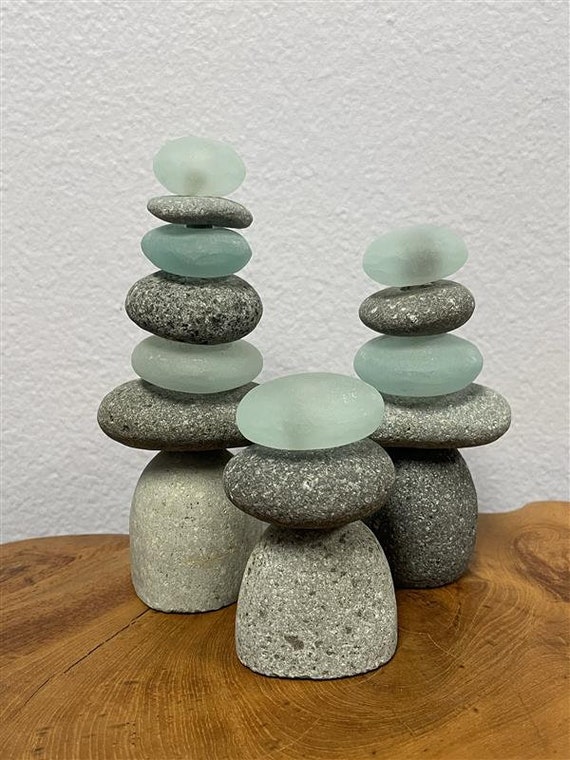The image captures a detailed arrangement of three towers of small, stacked stones on a wooden tabletop. The tabletop is made from a live edge cut of wood, showcasing the intricate grain and core of the tree. The stones vary in color, including light gray, dark gray, and light teal, with a slightly see-through, foggy appearance. The front stack, consisting of three stones, is the shortest. Behind it are two taller stacks; one has seven stones, and the other has five. The stones, resembling pebbles with a unique base stone different from the others, appear to be held together by a dowel. The scene is set against a white wall, providing a serene and artistic display.